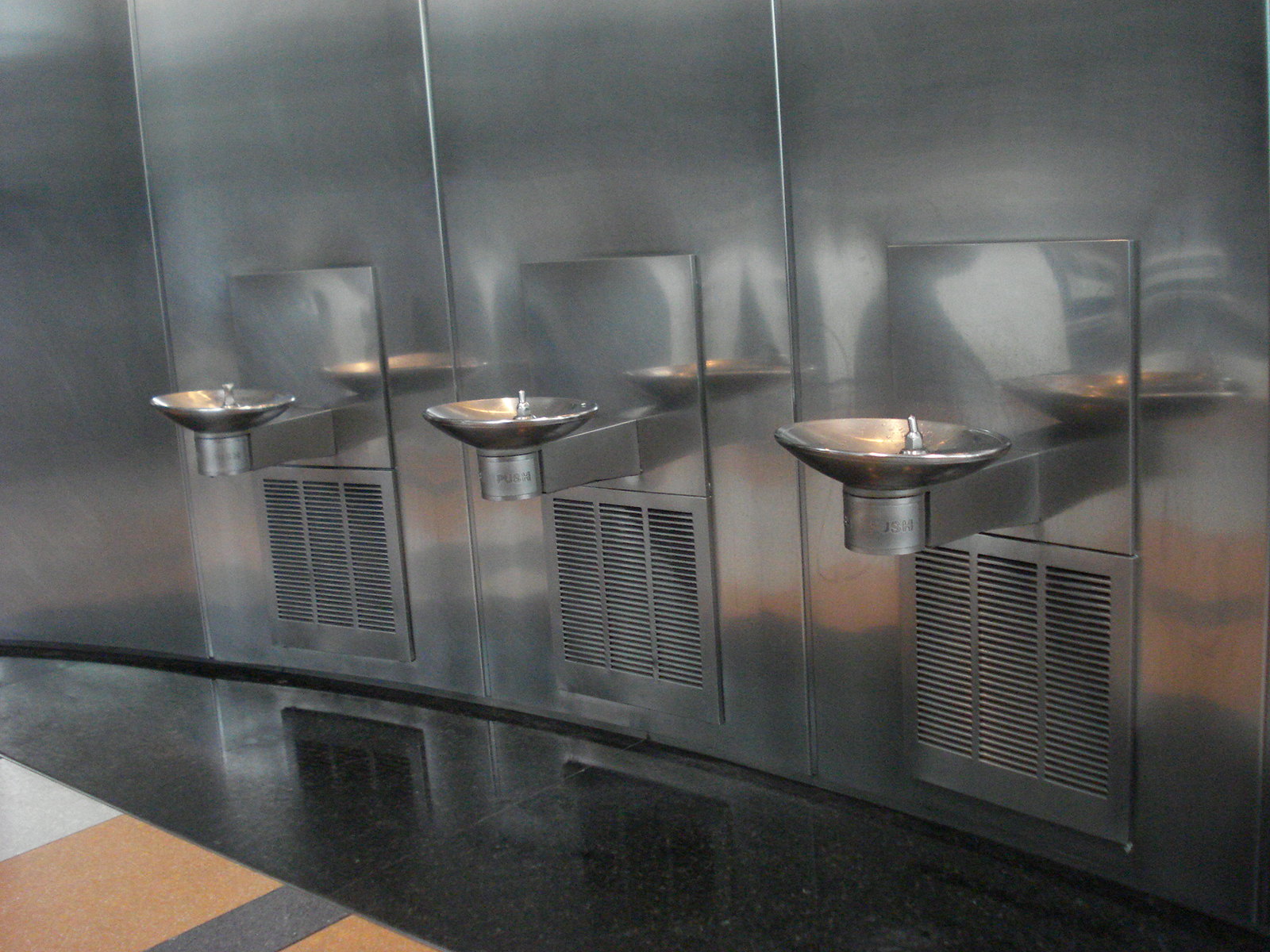This image captures a section inside a building where three water fountains are mounted on a slightly curved, stainless steel wall with a silver brushed finish that resembles the sleek exterior of an Airstream trailer. Each water fountain features a round, basin-like design with a silver nozzle emerging from the right side. Below each fountain, the wall has vent openings in groups of three, separated by a vertical line. The floor is a shiny, possibly granite tile, transitioning into a dark gray semicircular design, which then blends into an orange, white, and light gray pattern toward the lower left corner. To the left side of the image, there appears to be a main hallway, suggesting that these fountains are conveniently placed in an inset metallic alcove for easy access by passersby seeking a quick drink of water.